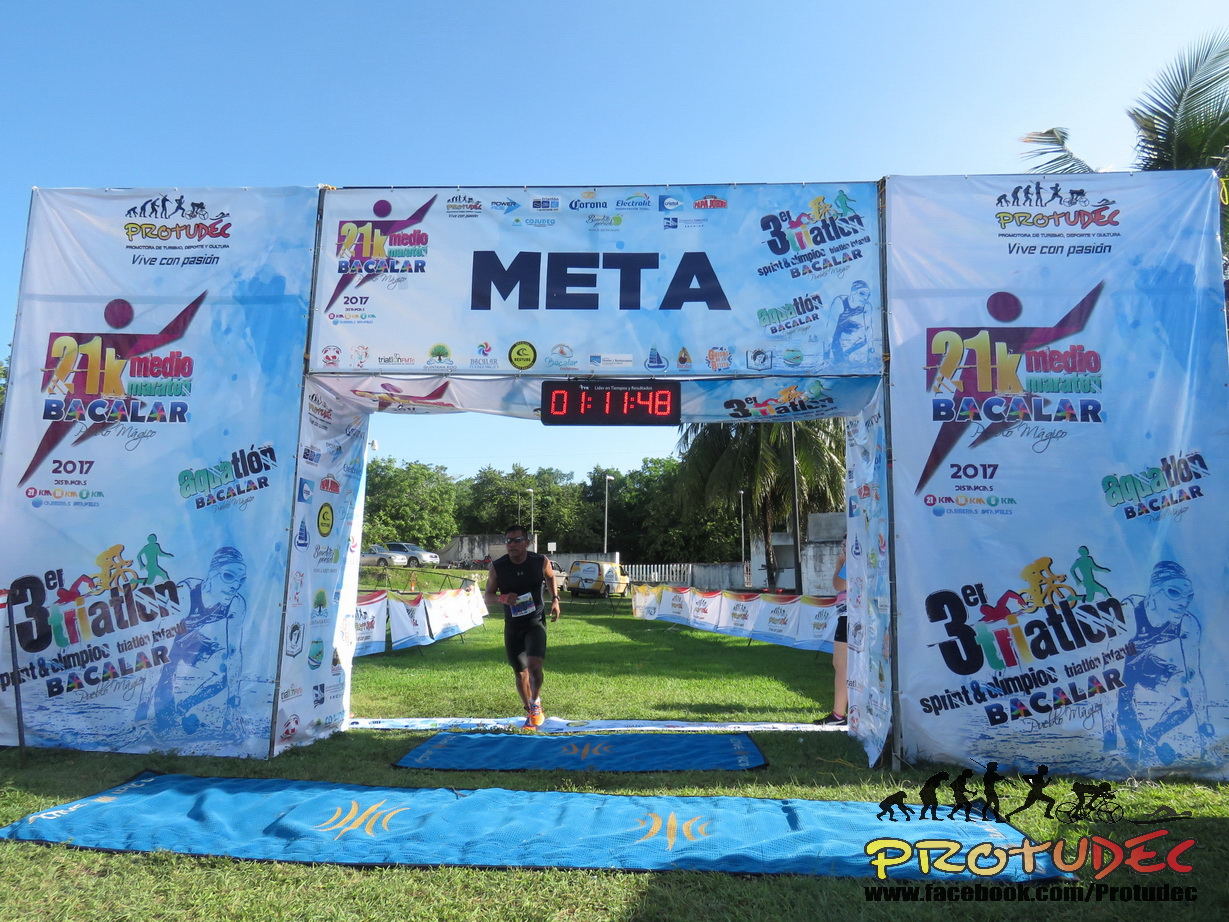In this vibrant image, a runner clad in black and sporting sunglasses is captured just as he crosses the finish line of the 21K Medial Marathon Bacalar, held in what appears to be a scenic, grassy area adorned with palm trees and other vegetation. The finish line is marked by a white arch assembled from metal rods and draped with colorful tarps and banners, collectively forming a tunnel-like structure. Dominating the arch is the large, bold word "META," and beneath it hangs a digital clock displaying a race time of 1 hour, 11 minutes, and 48 seconds in bright red numerals.

The arch and surrounding area are festooned with various logos and pieces of artwork, adding splashes of vivid color. Among these is a Pro2Deck logo, featuring a gradient from yellow to red and depicting an evolutionary progression from monkeys to modern athletes. Another prominent logo includes a stick figure in a dynamic running pose. The event is heralded as the 21K Medio Bacalar and includes references to a triathlon, such as the L3 Triathlon Bacalar and Aquation Bacalar, indicating multifaceted athletic events like running, biking, and swimming.

Beneath the finish line arch, a blue mat extends across the ground, flanked by another mat adorned with yellow logos, welcoming the runner as he completes his race. To one side, the banners forming the race chute guide the participants. In the background, cars and an additional figure are visible, adding depth to the scene. Pro2Deck’s logo and web address (www.facebook.com/Pro2Deck) are prominently displayed, emphasizing the event's sponsors.